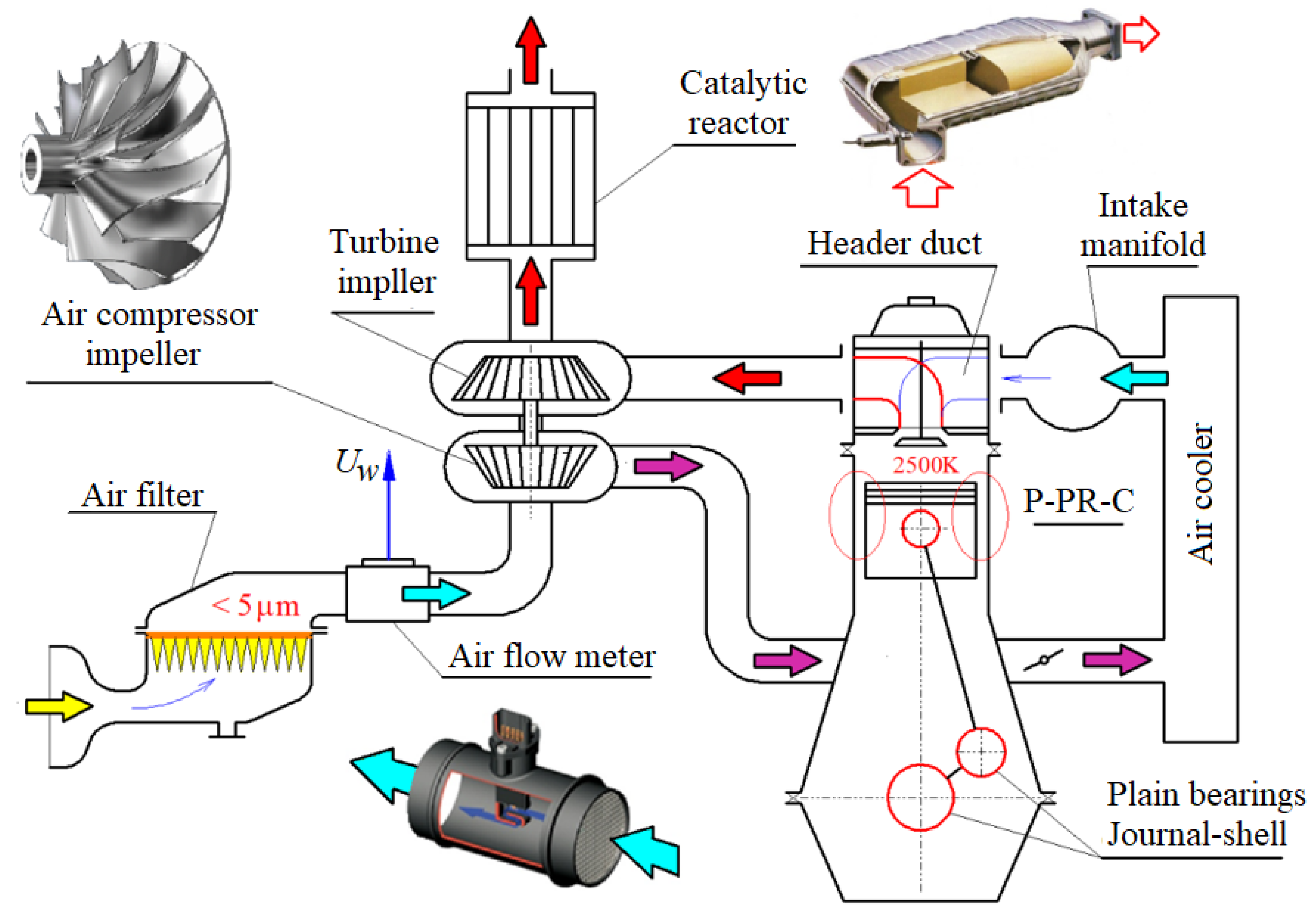This comprehensive computerized schematic illustrates the intricate workings of an engine, highlighting key components and their interactions with detailed colored annotations. In the top left, we find a black and white sketch of an air compressor impeller marked in red text, transitioning to an air filter denoted with a yellow arrow pointing right. Below, a purple arrow traces the path to a turbine impeller, indicated by red arrows pointing upward. The schematic continues to the air flow meter and moves rightward to reveal the catalytic reactor and the header duct. The header duct guides air past the air cooler, outlined with a light blue arrow, moving towards the intake manifold. At the bottom right, we see the plain bearings journal shell, typically found on a crankshaft, explained as a piston rod clamped around a bare shaft without intervening ball bearings. Noteworthy features include several colored arrows, such as a red arrow illustrating the flow from the turbine impeller towards the catalytic reactor. The intake manifold and air cooler show a sequential flow of air, crucially marked with purple and light blue arrows, visualizing the air’s journey through the engine’s intricate system.